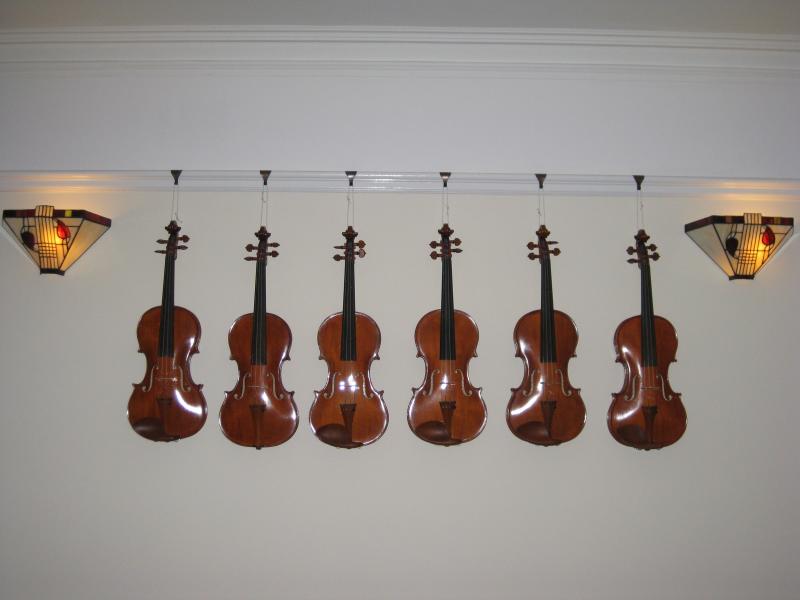The photograph depicts a set of six identical violins, each with a black neck and dark brown, walnut-colored body, hanging from strings attached to black hooks on a cream-colored wall. The wall features white wainscoting near the top, blending seamlessly with the crown molding. The violins are symmetrically arranged between two Tiffany-style wall lamps, positioned about a third of the way from each edge. These lamps, shaped like inverted pyramids, display etchings of birds and possibly fruit like apples and grapes in green and red hues, with a pattern of vertical and horizontal lines. The violins dangle gracefully between these light sources, adding a touch of musical elegance to the well-lit and carefully detailed wall space.